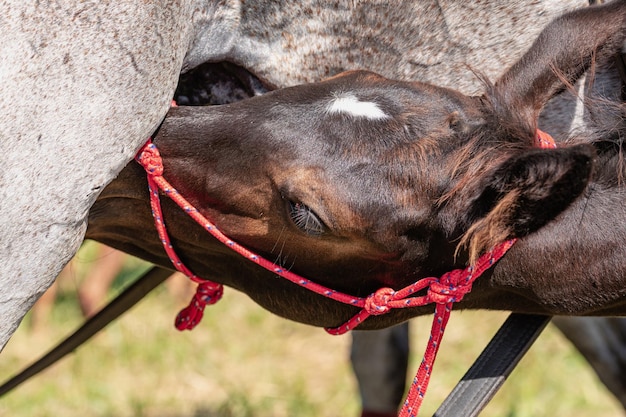The image captures a young foal, a dark brown horse with a distinct white patch on the top of its head and long, pointy, dark brown ears. The foal is adorned with a red rope, speckled with blue, around its neck and face area. It appears to be nursing from its mother, whose lower body and light tan color with possible gray specks are partially visible. The foal is reaching up to its mother’s udder in a close-up shot. They are outside, surrounded by muted green grass and possibly a fence, under a clear sunny sky.